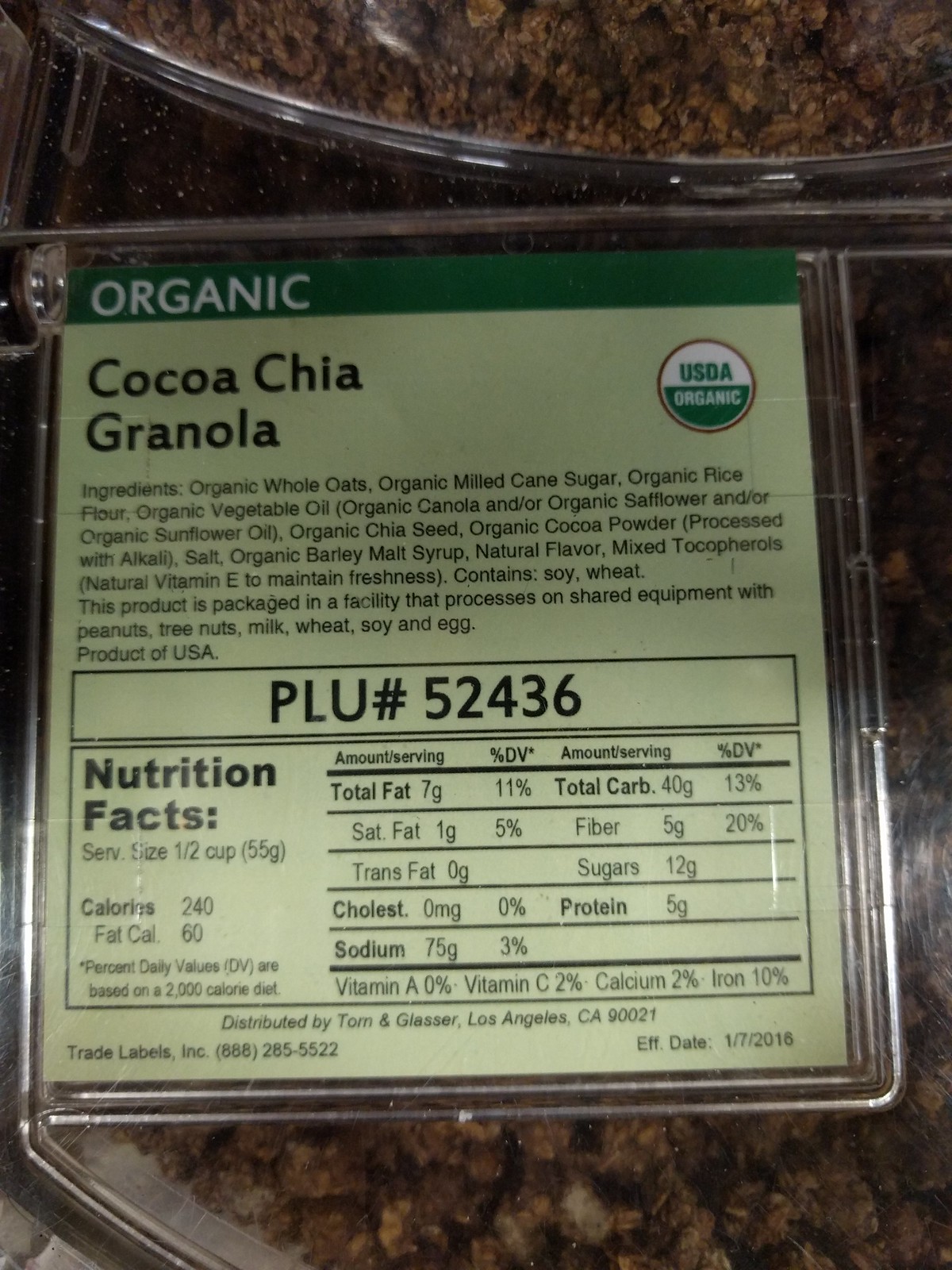The image showcases a bulk container of chocolate chia granola with a detailed ingredient list and nutrition facts label. The granola is stored in a large plexiglass bin, and customers can dispense their desired amount into a bag, weigh it, and pay. 

A paper or cardboard card inserted into a plastic holder displays the information. At the top, a green bar prominently marks the product as "organic." Behind the card, you can see the granola, a mixture of various ingredients.

The ingredient list includes: organic whole oats, organic milk, cane sugar, organic rice flour, organic barley malt syrup, natural flavor, and mixed tocopherols. The product is made in the USA and is processed in a facility that shares equipment with peanuts, tree nuts, milk, wheat, soy, and egg.

The nutrition facts label indicates that a half-cup serving (55 grams) contains 240 calories, with 60 calories from fat. Notably, there is an error on the label: it states 75 grams of sodium, which should be 75 milligrams, equating to 3% of the recommended daily value.